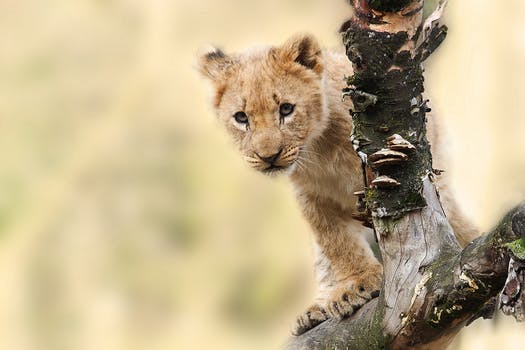A curious baby tiger cub with dark eyes and small ears is perched on a tree branch in front of a washed-out, light yellow backdrop. The cub's fur is an orange-ish white, soft and fluffy, indicating its young age, possibly three to four months old. It stands on all four paws, which appear proportionally large, behind a vertical branch that bifurcates from a diagonal one. The tree it's on is adorned with green moss and shelf-like fungi. The fungi, common in wooded areas, are known for their potential use in fire starting when processed. The background is blurred, emphasizing the cub's focused, inquisitive gaze directed straight at the camera.